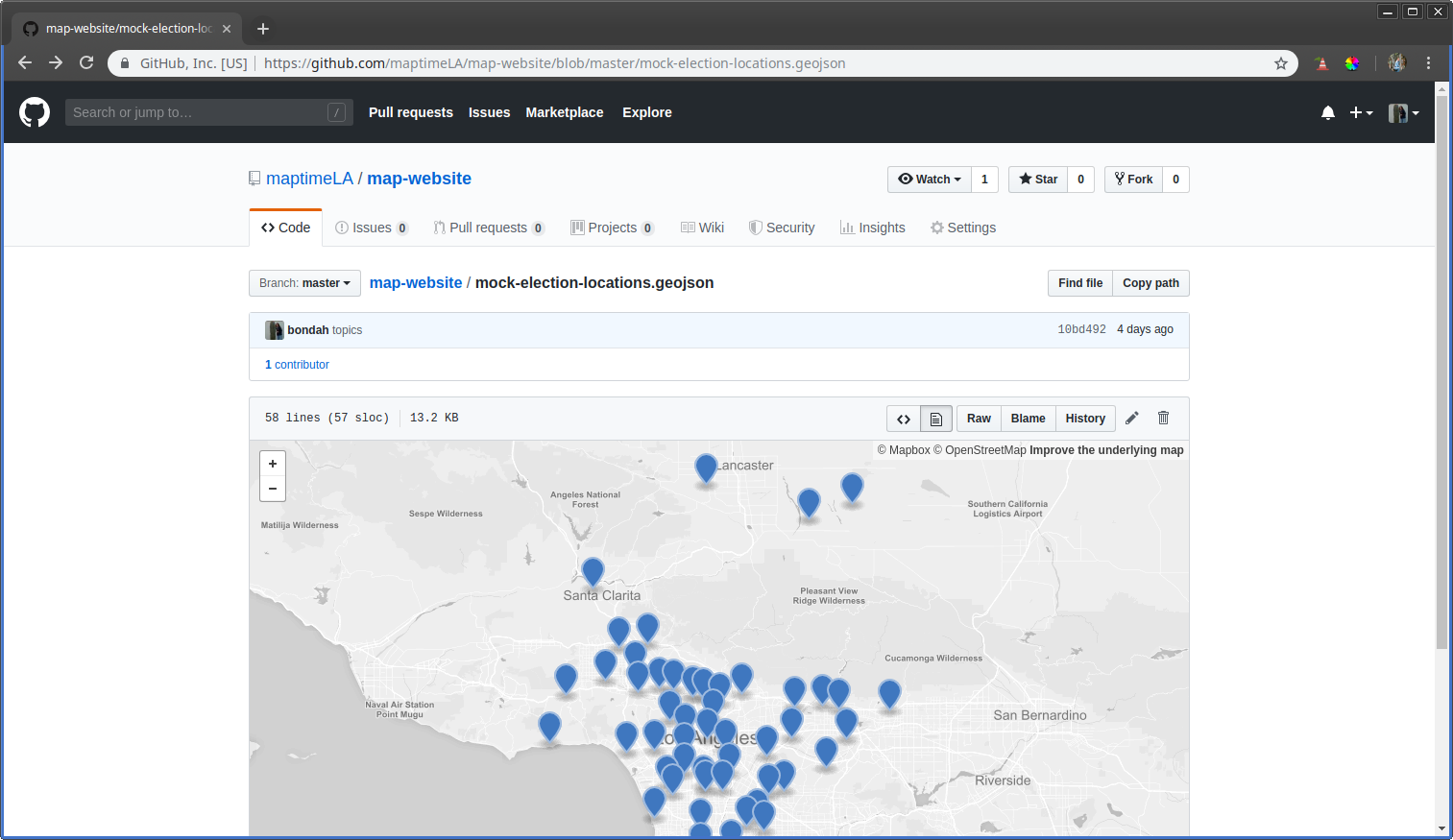This screenshot captures a webpage displayed on a computer screen, identified as the MapTime LA site, specifically the "map-website" section. The browser interface is visible, including a tab in the upper left and a search bar across the top. The main content features a grey map with numerous blue location dots concentrated mostly south of Santa Clarita and a few around Lancaster in the top center. The bottom right of the map also highlights the areas of San Bernardino and Riverside. 

The webpage has a white background, and beneath the MapTime logo, navigation options are listed including 'Code' (the selected tab), 'Issues,' 'Pull Requests,' 'Projects,' an unreadable entry, 'Security,' 'Insights,' and 'Settings.' Additionally, within the webpage hierarchy is the path "map-website/mock-election-locations-geojson."

On the left-hand side, there is a small profile picture and a name, though the name is not legible in the screenshot.